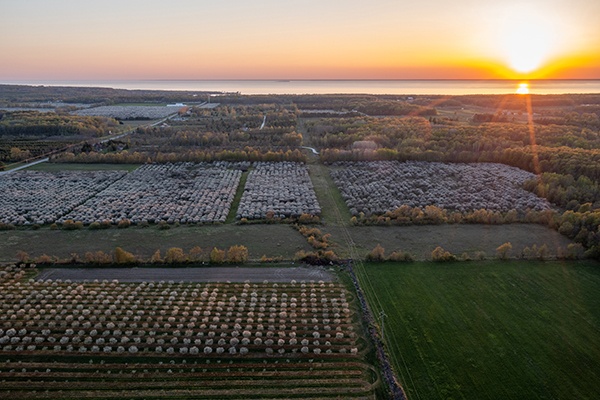This aerial photograph captures an expansive farmland that stretches as far as the eye can see. The fields are meticulously organized into neat rows populated by large, white, bushy-looking plants, possibly resembling cotton or some type of rolled-up harvest. Each row is flanked by green pathways that provide a striking contrast to the white crops. The fields are divided by thick strands of green grass and lines of trees, adding to the orderly landscape. Running centrally through the image are telephone poles that extend straight into the distance.

Surrounding the fields, there are various clumps of dense, green forest trees. At the top section of the image, toward the right-hand corner, the orange sun is setting, casting a warm glow that suggests the photograph was taken at dusk. Further in the background, a large, calm body of blue water is visible, adding a serene element to the rural scene. The image appears to have been taken from an elevated vantage point, possibly 100 to 200 feet up, providing a comprehensive view of the diverse and picturesque landscape below.